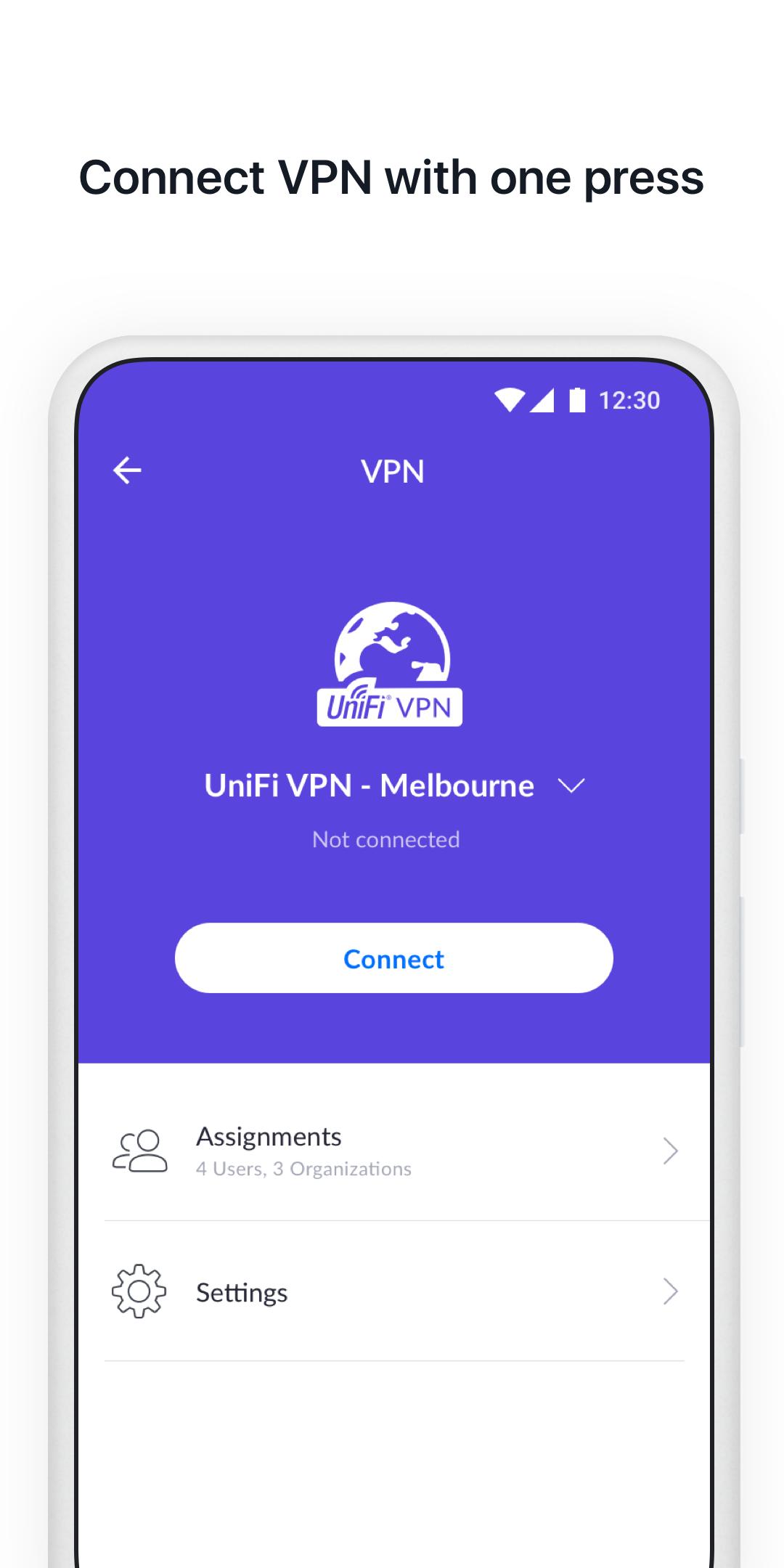The website advertises a VPN service with a clean, modern design. At the top, a bold black heading reads "Connect VPN with One Press." Below, there's a mockup of a smartphone screen designed to demonstrate the app's interface. The surrounding area is mid-gray, while the smartphone display draws attention with a large, purple rectangle occupying approximately two-thirds of the screen space. 

On the left side of this rectangle is a bold white arrow pointing left, and centrally positioned, the acronym "VPN" is displayed prominently in bold white text. The status bar at the top of the mockup shows full WiFi, cellular signal, and battery icons, accompanied by the time "12:30," suggesting a 24-hour format.

A striking image of the Earth features purple oceans and white landmasses, next to which is a WiFi symbol inside a gray rectangle with a purple border. The text within reads "Unify (UNI, FI™) VPN." Below this, but outside the rectangle, "Unify VPN - Melbourne" is written along with a checkmark, indicating the selected server location, and the status "Not Connected" in gray text.

Towards the bottom is a clickable oval button in light gray with cyan blue text. The interface also includes two silhouette icons labeled "Assignments" in black, with subtext in gray denoting "4 users, 3 organizations" accompanied by a right-facing arrow. Finally, a gear icon is labeled "Settings" in bold black with a gray arrow beside it.